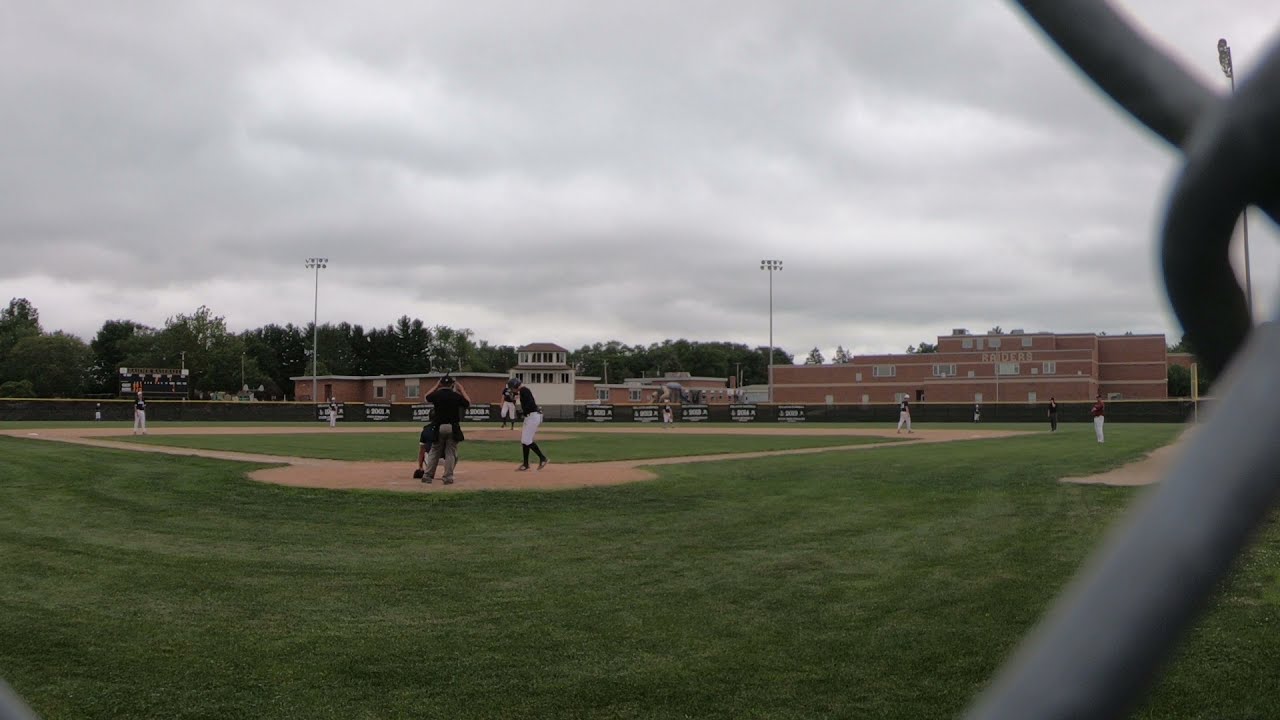This full-color landscape photograph captures an overcast day at an outdoor high school or college-level baseball game. Taken from ground level through a chain-link fence visible on the right edge, the scene is viewed from behind the batter, umpire, and catcher as the left-handed batter approaches home plate. The meticulously maintained green grass contrasts with the red dirt outlining the bases. Various players are scattered across the field, with the umpire facing away from the viewer. In the background, an empty field stretches out under a threatening gray sky, suggesting imminent rain. The distant horizon features a scoreboard, several large floodlights, and a red multi-story brick building. There are no visible residential areas or parked cars, further indicating the isolated park-like setting of the game.